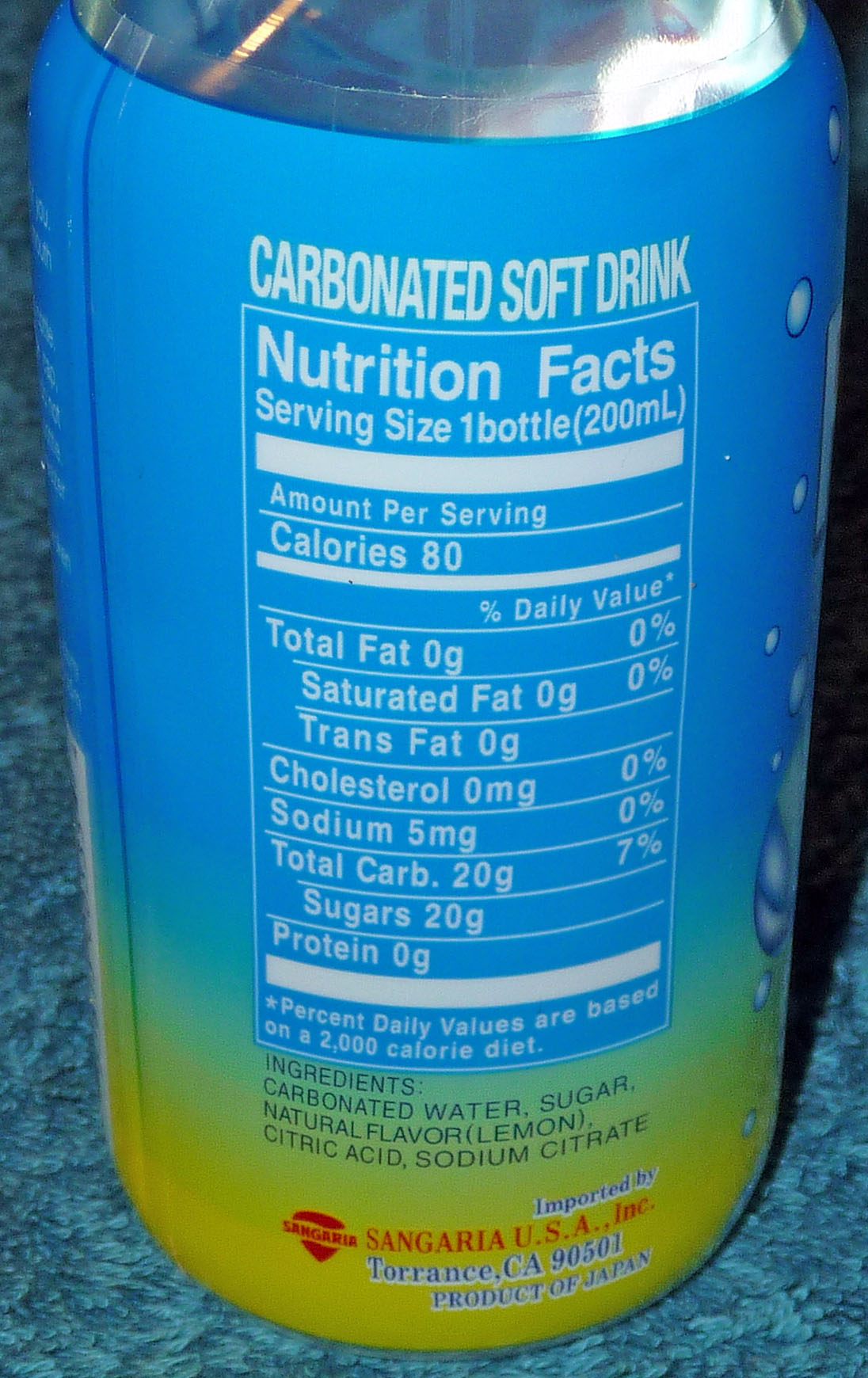The image showcases a bottle featuring a vibrant and detailed label. This label belongs to a carbonated soft drink, a popular beverage. The design transitions smoothly from a striking blue at the top, through a greenish gradient, culminating in a bright yellow at the bottom, likely to attract attention and suggest a refreshing flavor profile. The label indicates that the product is an imported beverage from Japan, distributed by Sangaria USA Inc., located in Torrance, California, 90501.

Nutritional information for the 200-milliliter serving size is clearly listed. Each serving contains 80 calories, with no trans fat, saturated fat, or total fat. It also has zero cholesterol, 5 milligrams of sodium, 20 grams of total carbohydrates (7% of the daily value), 20 grams of sugars, and no protein. The drink’s ingredients include carbonated water, sugar, natural lemon flavor, citric acid, and sodium citrate.

This detailed composition and visually appealing label make it a notable example of how beverages can attract consumers through effective packaging design and clear nutritional labeling.